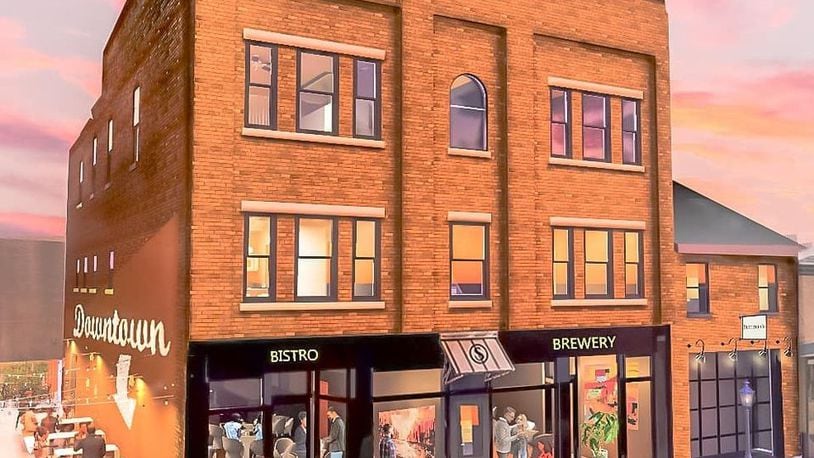This detailed and illuminated image captures an artistic representation of a three-story brick building situated in a downtown area. The building, constructed in an old brick industrial style, showcases a series of windows. These include four sections of three rectangular windows each on the top floors, flanking two smaller central windows, one of which features a rounded arch. The vibrant sky in shades of pink, orange, and blue — resembling a sunset — forms a striking backdrop. 

Emphasizing the artistic nature, the image is viewed from an aerial perspective, with the ground obscured. Prominently displayed on the left side of the building is a bold sign with the word "DOWNTOWN" accompanied by a downward-pointing arrow. This side also has an outdoor seating area with visible tables and patrons.

On the main floor, the building houses a restaurant and brewery, marked by two signs: "Bistro" on the left and "Brewery" on the right. Below these signs, an awning extends beneath the central windows. Visible inside through the ground floor windows, various people can be seen, adding life and activity to the scene. The juxtaposition of these architectural details against the colorful sky and bustling ground level creates a comprehensive and vivid depiction of the downtown building.